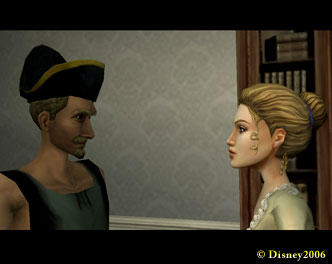This computer-generated image, likely from a game or show, is framed with a black trim at the top and bottom, but none on the sides. In the bottom right corner, the text reads "© Disney 2006." The scene features a man and a woman engaged in conversation. 

The woman, positioned on the right, has her brown hair styled in a bun and wears a green blouse adorned with white frilly trim. She is facing the man to her left. The man, on the left side, faces the woman. He sports a black hat with gold trim, has brown hair, and a long chin. His attire includes a tank top-style shirt, primarily green with black edges. 

The background consists of wallpaper with a white piece of trim near the bottom. Additionally, behind the woman on the right, there is a bookshelf filled with books, adding depth and context to the setting.